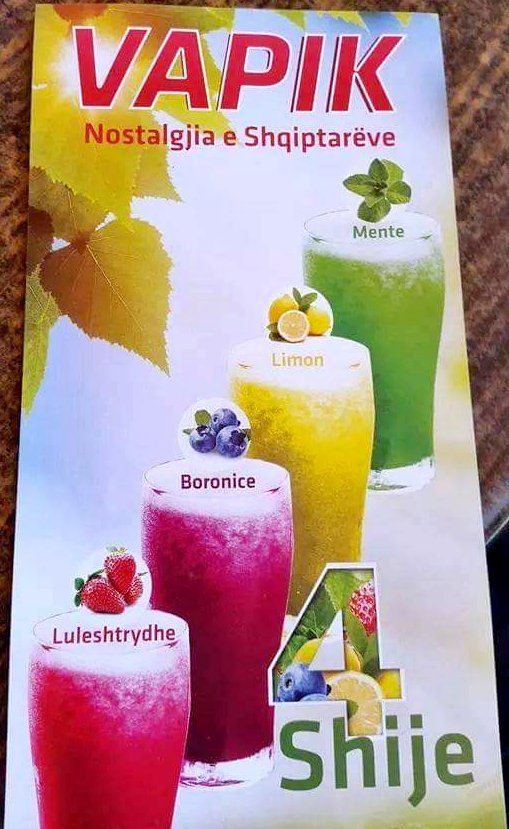The advertisement is for a product called "VAPIK Nostalgia E Shqiptareve," prominently displayed in bold red text at the top of the flyer. The backdrop of the flyer is predominantly white, enhancing the visibility of the vibrant details. In the upper right corner, there's an illustration of sharp, jagged yellow leaves with a central vine, signifying autumn, with the sun shining behind them and a glimpse of blue sky above. Below the title, arranged vertically, are four tall glasses filled with colorful drinks. From left to right, the first glass contains a red strawberry drink labeled “Luleshtrydhe,” adorned with a fresh strawberry. Next is a deep reddish-purple blueberry drink labeled “Bornonice,” topped with blueberries. The third glass is a bright yellow lemon drink labeled “Limon,” garnished with a lemon slice. The fourth is a green mint drink labeled “Mente,” with a sprig of mint on top. The bottom right of the flyer features the number four in bold, outlined in white, surrounded by illustrations of strawberries, lemons, blueberries, and mint leaves, with the word “Shije” in green lettering beneath it.